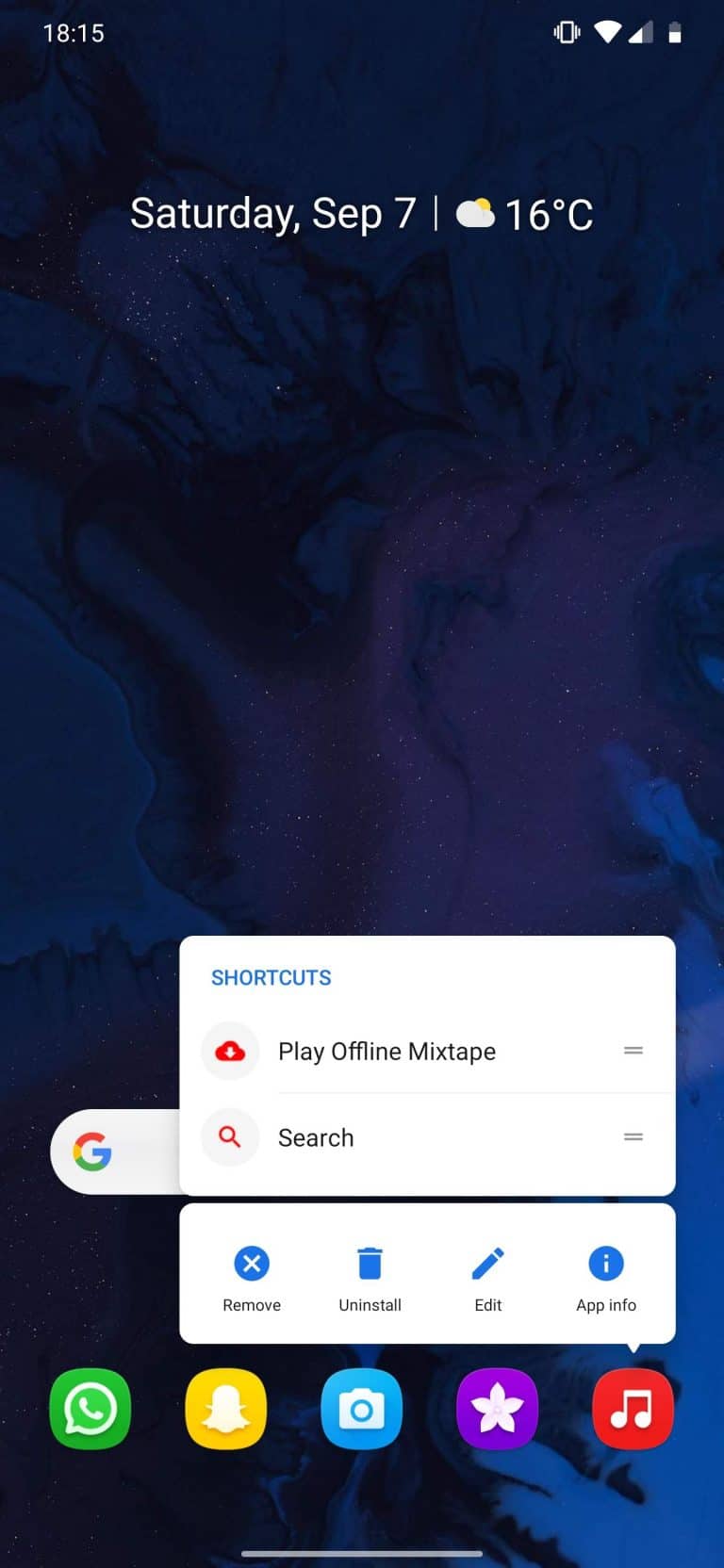In this vibrant image, a blue-black gradient forms the canvas, with intricate blue patterns dominating the top section and transitions through purple hues towards the bottom. The lower right corner features lighter blue patterns set against the black background. 

At the top left corner, the screen displays the time "18:15", accompanied by several status icons: a rectangle flanked by small knobs, a Wi-Fi symbol, a white triangle beside a gray bar, and a partially filled battery icon. Below these indicators, the date "Saturday, SEP 7" is displayed, with a horizontal line underneath. The weather is shown with an icon of a cloud and sun, labeled "16°C".

Moving down the image, a prominent white rectangle hosts the word "Shortcuts" in blue. Inside this box, there is a graphical representation of a red cloud with a play symbol, labeled "Play offline mixtape". Adjacent to it is an unclear icon or number. Below this section, a red search icon resembling a magnifying glass is labeled "Search" in black. Another indistinguishable icon appears to the right.

Protruding from the white rectangle is a light gray tab adorned with the multi-colored Google 'G'. Beneath this, another white rectangle features several blue icons indicating various functions: a circle with an 'X' for "Remove", a trash can for "Uninstall", a pencil for "Edit", and an eye for "App Information". 

Below these, there is a concise arrangement of colorful square icons with rounded corners: a green square with a speech bubble and phone, a yellow square depicting a ghost, a blue square with a white camera, a purple square with a light purple flower, and a red square with musical notes. The bottom of the image concludes with a thin white line stretching across.